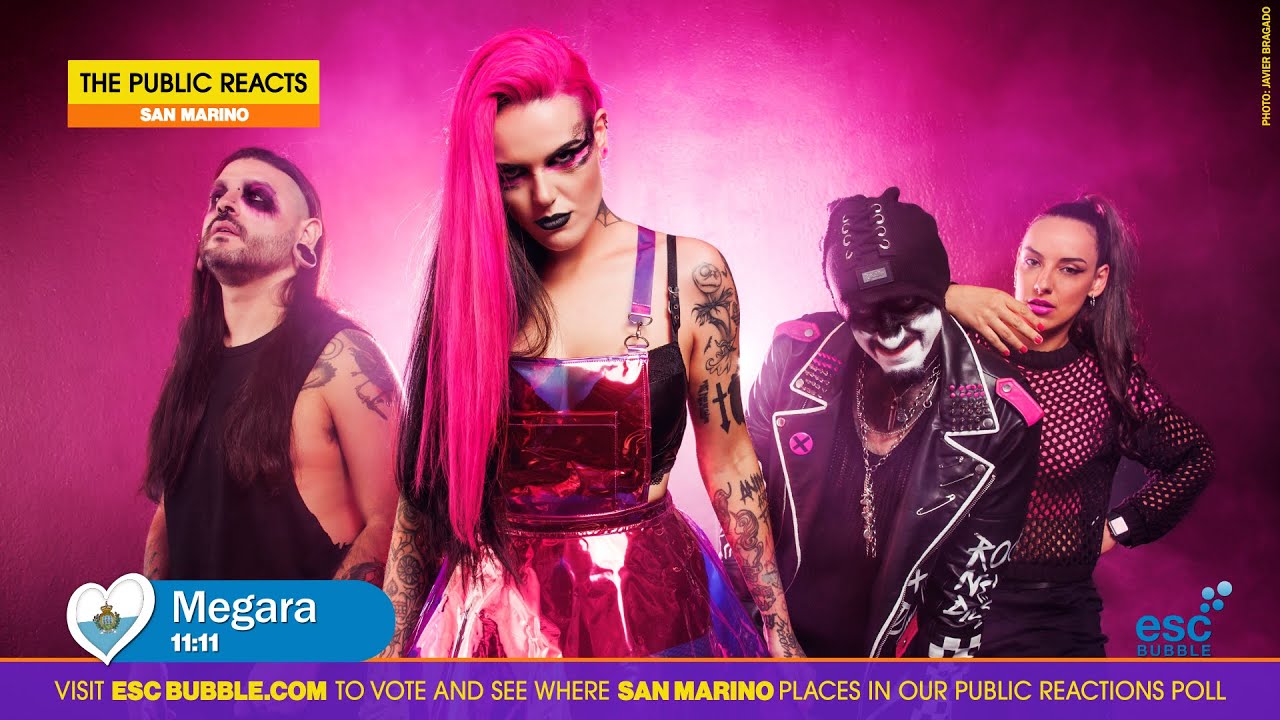In a striking pink-themed image, four individuals are featured against a bold pink backdrop. The upper left corner reads "The Public Reacts," while the bottom corner indicates "Megara." Additionally, a message at the bottom urges visitors to "visit escbubble.com to vote and see where San Marino places in our public reaction poll."

On the left stands a man with long hair cascading down his shoulders, adorned in black eye makeup. His sleeveless shirt reveals a tattoo on his arm, and he gazes pensively upwards and to the left. Beside him is a woman dressed in a vibrant, vinyl-like pink dress. Her long, pink hair complements her serious expression as she looks straight ahead, showing off the tattoos on her arm.

Next to her, a man with a tuxedo-patterned shirt but no jacket stands with his head bowed down. His face is painted white, and he sports a hat. Tattoos cover his exposed torso. A woman beside him rests her arms gently on his back. Clothed in a mesh pink shirt, her long brown hair frames her impassive face as she looks directly into the camera.